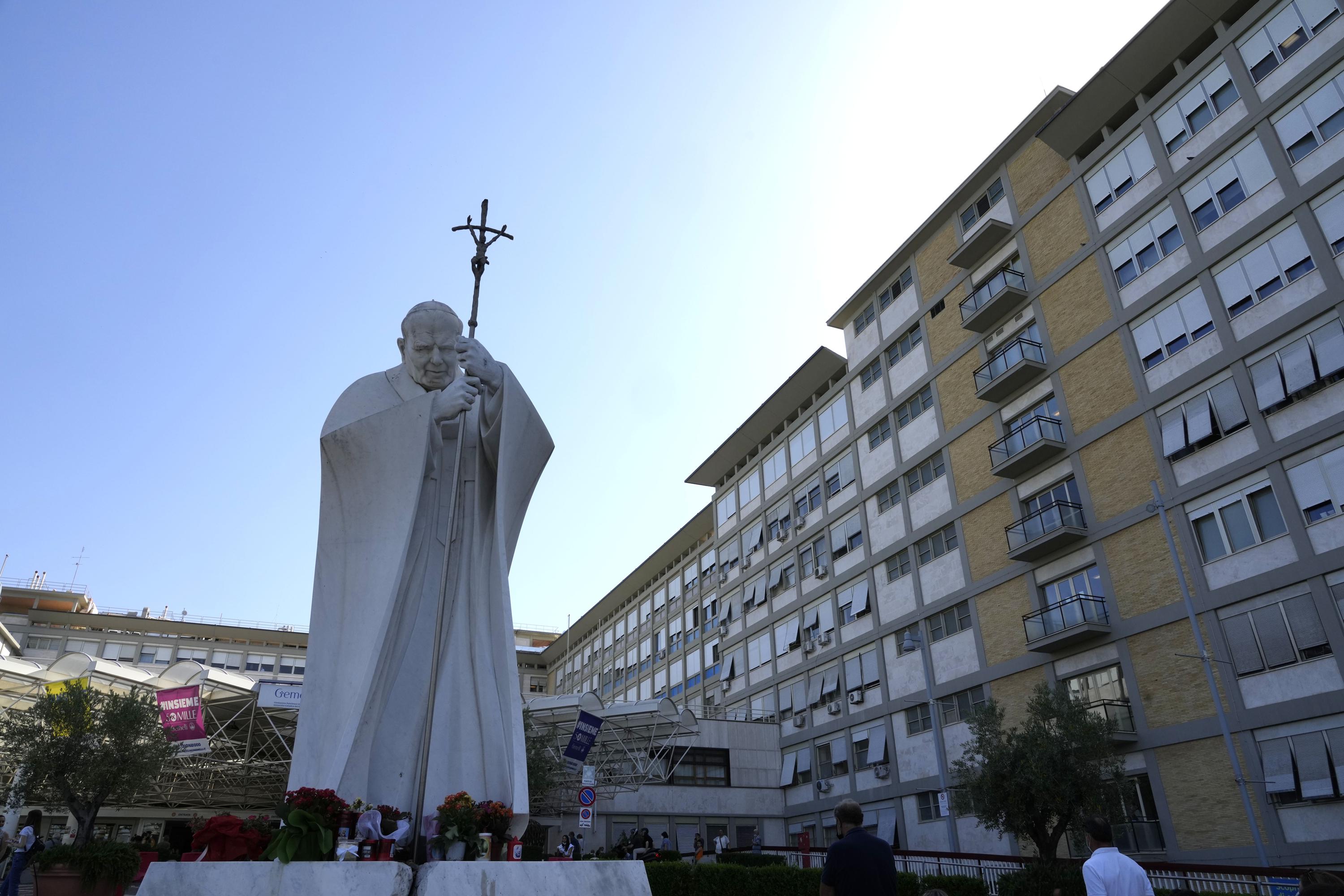The photograph captures a striking statue of a Catholic religious figure, presumed to be a Pope, standing prominently in the foreground on the left side. The all-white statue, adorned in robes, holds a tall scepter resembling a cross with a depiction of Jesus at its top. Behind this imposing figure, a sprawling apartment building wraps around, its numerous floors and windows varying between open and closed. Some windows have clothing or items hanging out to dry, and there are scattered balconies. People are seen walking on the ground, making their way to and from the building. Purple signs are partially visible behind the statue, although their text is unreadable. The scene is bathed in early morning light, casting a serene blue sky overhead and leaving the area beneath the building in shade. A small tree is noticeable within the courtyard area, adding a touch of greenery to the urban setting.